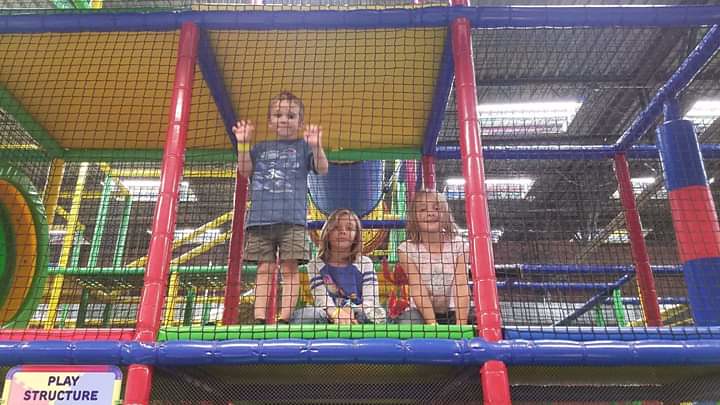The photograph captures the vibrant energy of an indoor play area, resembling a structure one might find at a Chuck E. Cheese. Central to the image are three children located in an elevated section of a colorful mesh-screened play structure. The structure itself boasts an array of colors with red vertical posts and blue horizontal bars, wrapped in soft padding for safety. The floor is a lively mosaic of red, green, and blue mats, while various tubes—some blue and yellow, others green and yellow—are visible in the background.

In the middle, a little boy stands out, his short brown hair catching the light as he smiles down at the camera. He wears a blue t-shirt paired with khaki shorts and has his fingers threaded through the netting, engaging directly with the viewer. Flanking him are two girls with shoulder-length blonde hair. The girl closest to him is also wearing blue— a striped baseball-style shirt and jeans—though her expression is less joyful, providing a contrast to her companion. The second girl, sitting to the far right, sports a simple white shirt and blue jeans, and she meets the camera with a cheerful smile. Capturing the essence of playful camaraderie, the scene is underscored by a small sign in the bottom right corner that reads "play structure."